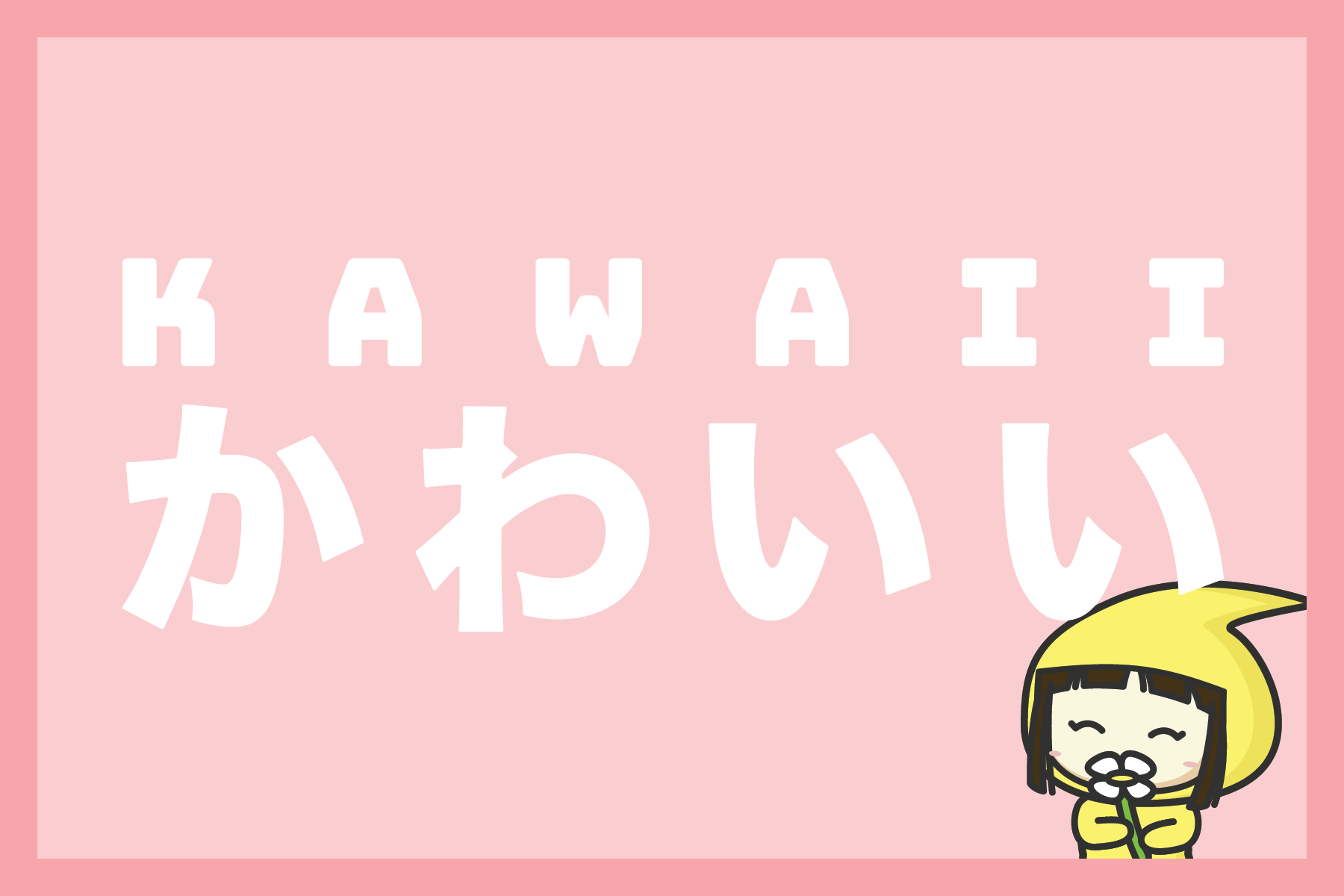The image is a cartoon-styled poster, depicted as a horizontal rectangle. It features a light pink interior with a darker pink framed border. Across the middle of the image, the word "Kawaii" is prominently displayed in large white capital letters, and beneath it are four Japanese kanji characters also written in white, which likely spell out the same word. In the bottom right corner sits a chibi anime-style character. She has a large head with fair skin, rosy cheeks, and closed eyes, suggesting a gentle expression. Her dark brown hair is styled with straight bangs and short, shoulder-length locks. She wears a yellow hooded outfit resembling a raincoat, with the hood shaped like a teardrop and pulled up. The girl holds a green-stemmed white flower close to her nose, appearing to sniff it softly.